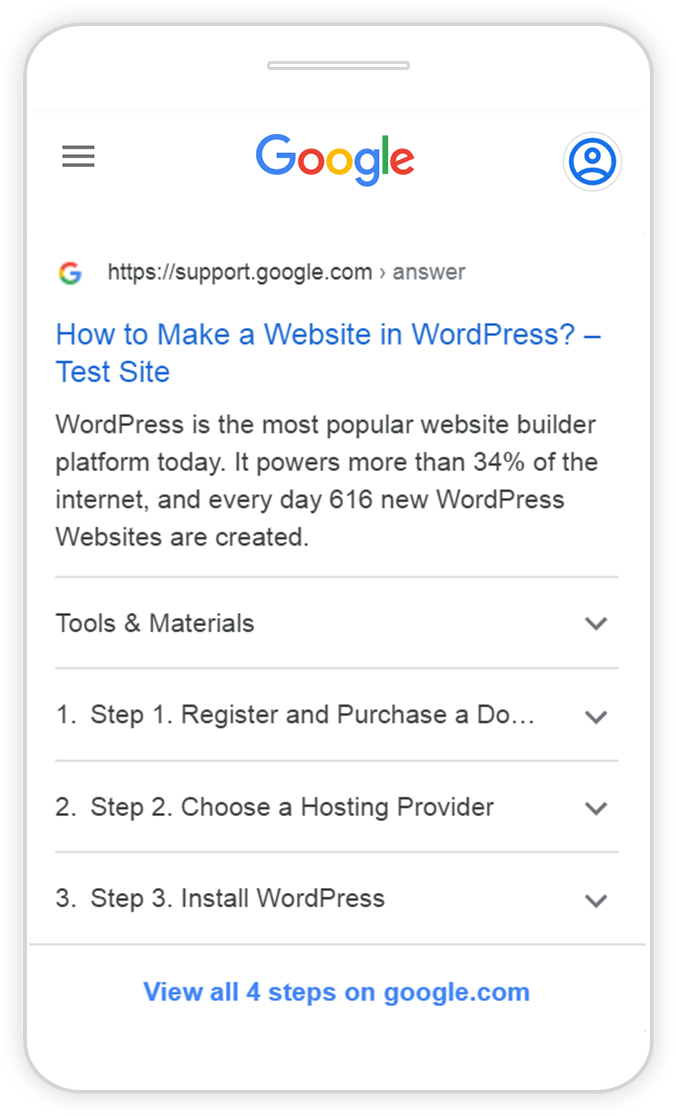In the image, the Google logo is prominently centered, featuring its signature colors of blue, red, yellow, and green. Below the logo, the URL "https://support.google.com/answer" is displayed. Under this, in blue text, the title reads, "How to make a website in WordPress? - Test site." 

Following the title, a paragraph in black text explains, "WordPress is the most popular website builder platform today. It powers more than 34% of the internet, and every day, 616 new WordPress websites are created." 

Beneath this paragraph, the heading "Tools and materials" appears, accompanied by a downward-pointing arrow. The step-by-step instructions follow:

1. Step one: Register and purchase a domain... 
2. Step two: Choose a hosting provider (with an arrow pointing downward) 
3. Step three: Install WordPress

At the very bottom, blue text invites viewers to "View all four steps on google.com."